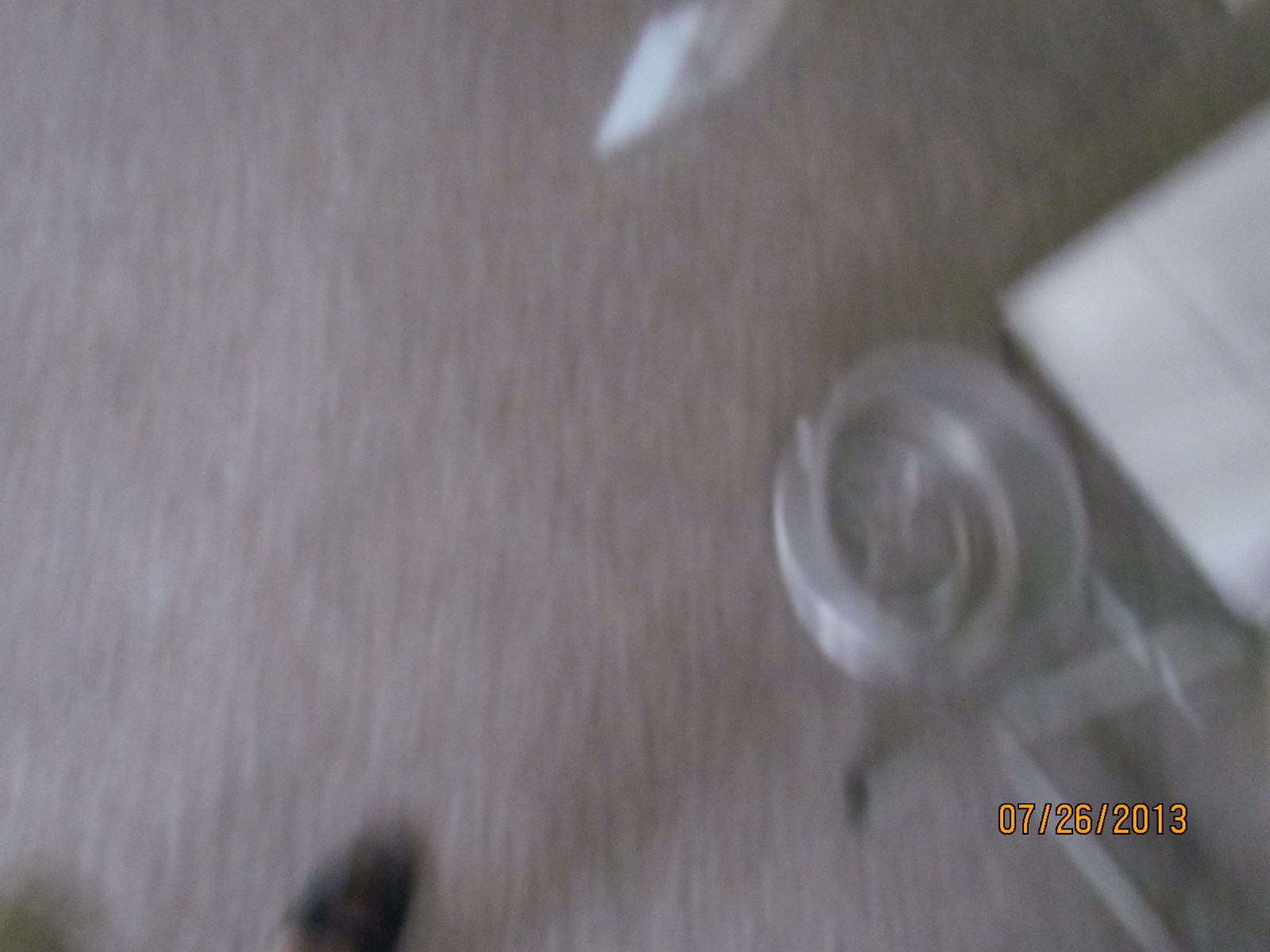A blurry, out-of-focus photograph captures an individual pointing their camera down towards a gray carpeted floor in an indoor setting. The rectangular image has shorter left and right sides compared to the top and bottom. Positioned in the bottom right corner, an orange timestamp bordered in black reads "07-26-2013." In the bottom left corner, the photographer's dark, almost blue, round-toed shoe and a portion of their tan-colored pants are visible. The right section of the image features an oval-shaped metal bowl or basket accompanied by a box.